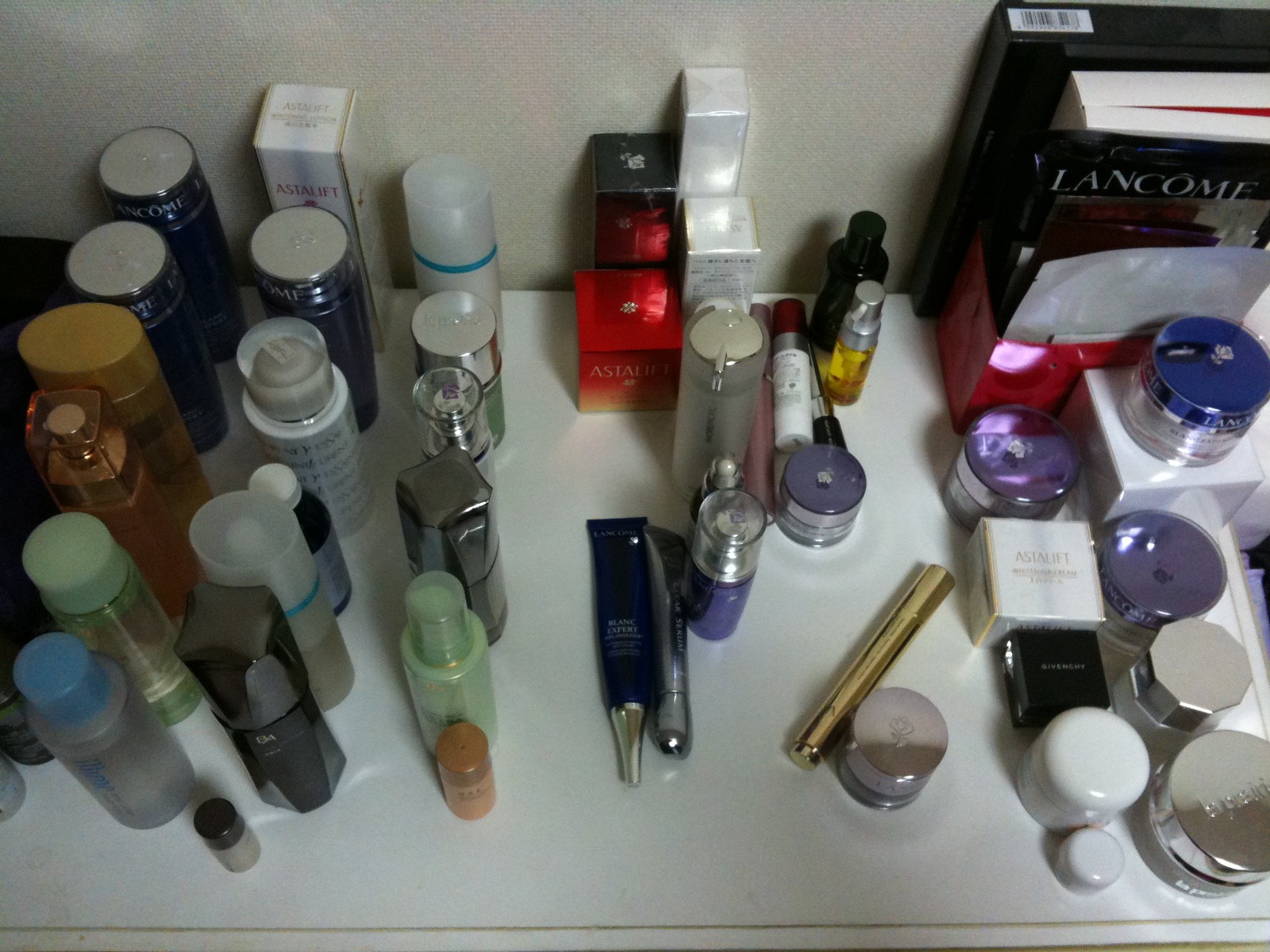The image showcases a meticulously organized desktop area set against a light gray wall and featuring a white surface. The surface is adorned with an array of cosmetics, skincare products, and books, creating a visually appealing display.

From left to right in the first row:
- Two blue bottles
- One golden bottle
- A golden spray bottle, presumably perfume
- A green bottle
- Another blue bottle

In the next row:
- A box labeled "Astylift"
- Another blue bottle from Lancome
- A white bottle
- A dark bottle
- A clear bottle
- Another perfume-like bottle with a small companion bottle beside it, possibly containing powder

Continuing along:
- A clear bottle
- A small green bottle with a metallic top
- Another perfume bottle
- A dark perfume-looking bottle
- A green bottle with another small bottle next to it

Lining the right side:
- Two medium-sized boxes and two large boxes with various cream tubes in front of them
- A purple container bottle

Further to the right:
- More cylindrical makeup-style bottles, including notable shades of yellow, black, and a small purple one
- A gold tube and a small silver bottle

Finally, an additional flat Astylift box is surrounded by:
- Purple containers
- A short Lancome branded bottle
- Several other containers with silver tops

All these items are neatly arranged next to an assortment of books, adding an organized yet vibrant touch to the desktop space.